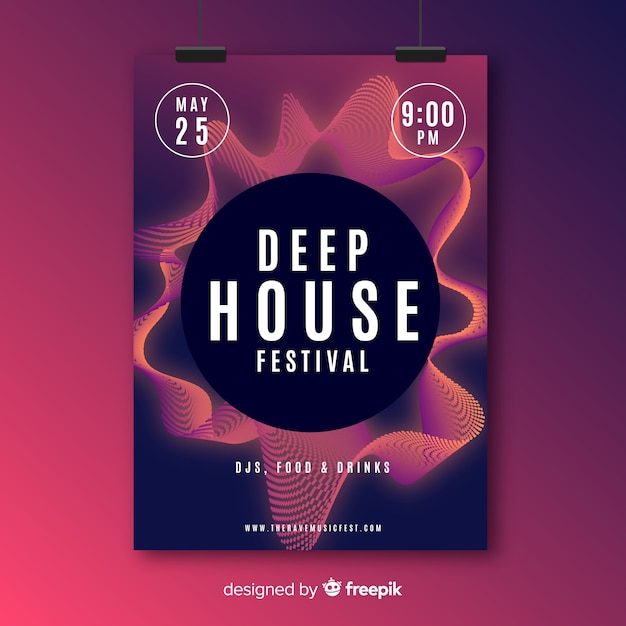This image is a detailed poster promoting the "Deep House Festival." The poster features an ombre backdrop that transitions from pink to purple. It is designed with symmetrically placed white circles in the upper left and right corners, detailing the date "May 25th" and time "9 p.m." respectively. The central focus of the poster is a large dark circle with contrasting white text that boldly announces "Deep House Festival," with the word "House" slightly larger than "Deep" and "Festival." Below this, in smaller white text, the poster provides additional details: "DJ's, Food and Drinks," followed by a web address, www.thesomethingmusicianstreet.com. The bottom of the poster also includes a white text acknowledgment: "Designed by Freepik." The backdrop features wavy light orange lines around the central circle, enhancing the visual appeal, and is further accentuated with varied purple and blue hues. The poster is secured by black clips at the top with a thin wire extending off the image, showing it is hanging against a wall that transitions from light purple on the left to darker purple and light pink hues around it.